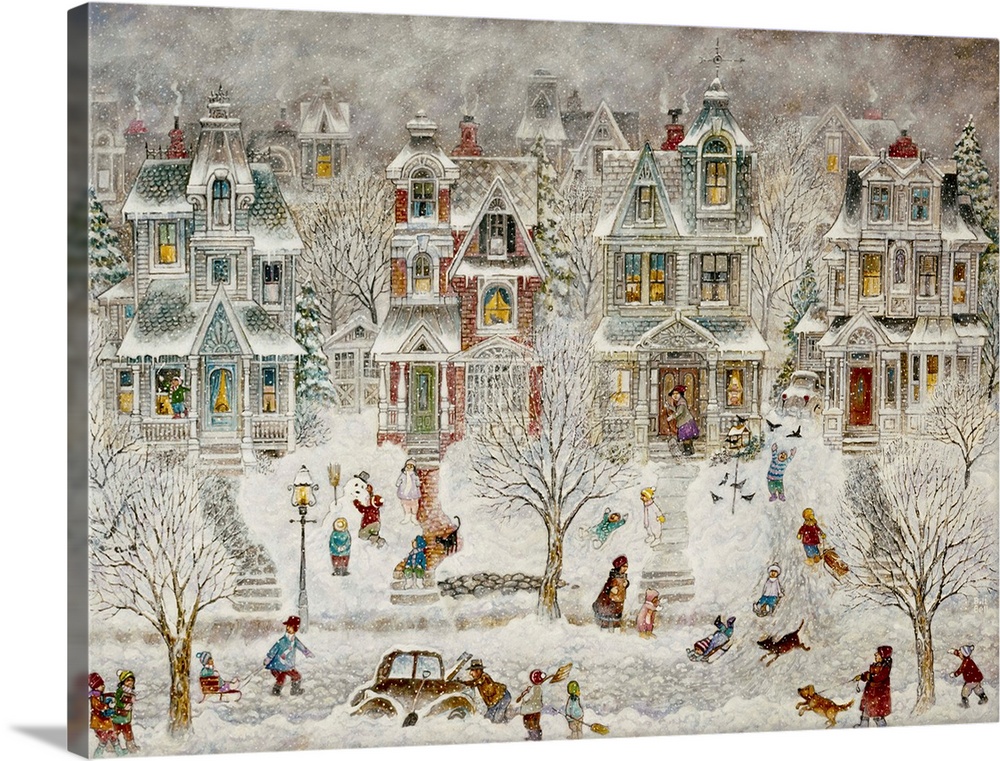The image depicts an idyllic winter scene, reminiscent of a canvas painting with a 3-dimensional effect that lends depth to the snowy setting. The view is of a city residential street, flanked by tall, three-story brick houses with sharply angled roofs, each covered in a blanket of snow. The scene is vibrant with activity: children are scattered throughout the yards, building snowmen, engaging in snowball fights, and taking turns sledding down driveways. The street itself is a flurry of white, peppered with scattered footprints and tire tracks.

In front of the houses, a car is stuck in the snow, with three people attempting to free it—one person with the hood up, another wielding a shovel, and a third holding a broom. Dogs play exuberantly in the snow, one on a leash held by a nearby woman. Leafless trees, coated in ice, stand in various corners of the image, adding to the wintry atmosphere. The entire scene is rendered in shades of white and grey, adding to the dreamy, almost storybook quality of this winter landscape.